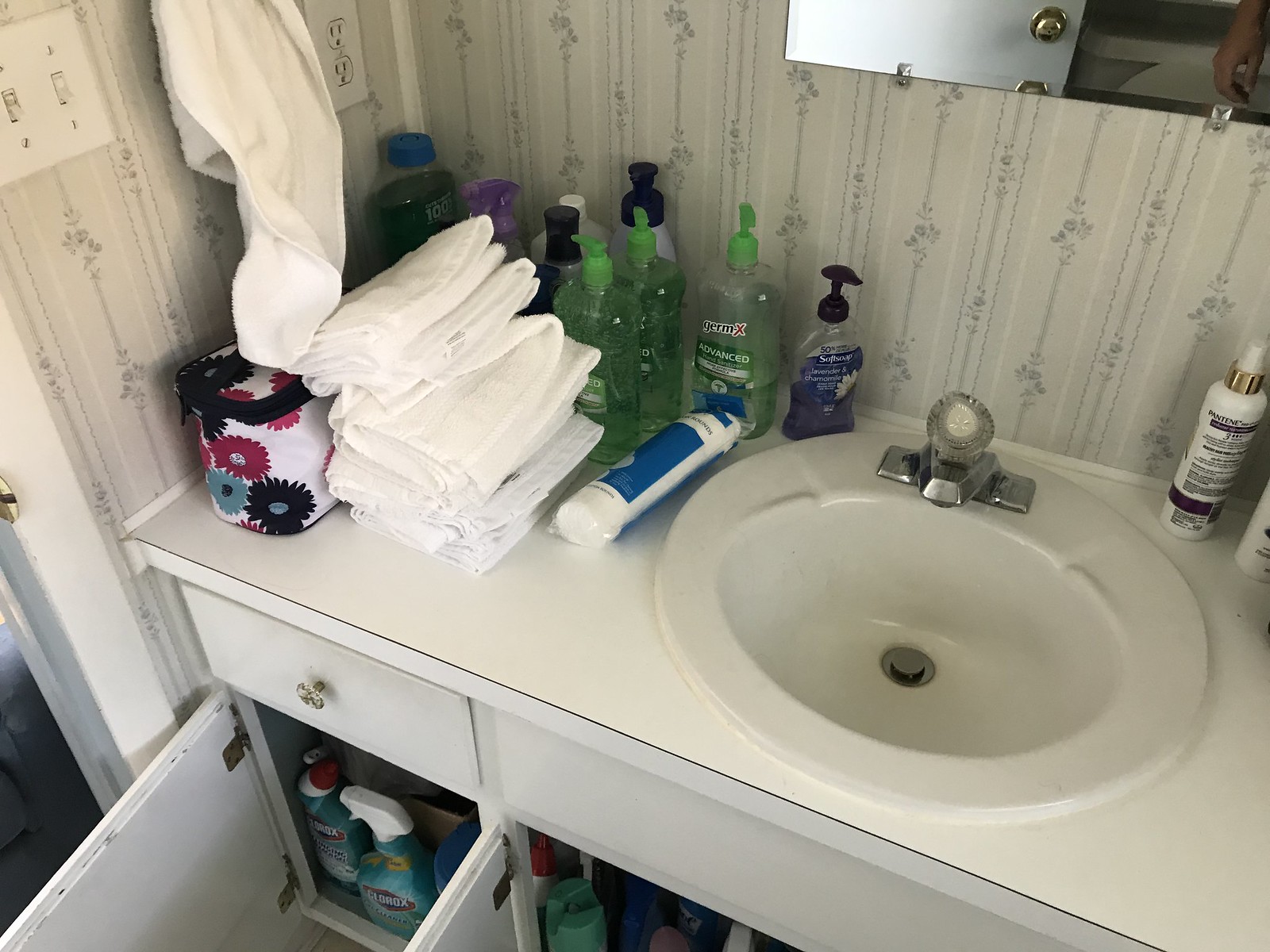The image features a pristine white wall accented with a delicate, elegant design. Centrally positioned against the wall is a sleek, silver faucet with a single-knob mechanism. Attached to the faucet is a thin, silver chain, contrasting subtly against the fixture's metallic sheen. Below, a set of cabinets, distinguished by their clean lines and minimalist design, house a variety of items. On the top right of this cabinetry, various spray bottles are neatly arranged. Above the faucet area, a mirror captures the partial reflection of a person's hand. Additionally, an assortment of toiletries is visible, including several bottles of green soap, a shampoo bottle, and a white-and-blue colored bottle. Hanging towels add a touch of softness to the overall streamlined aesthetic.